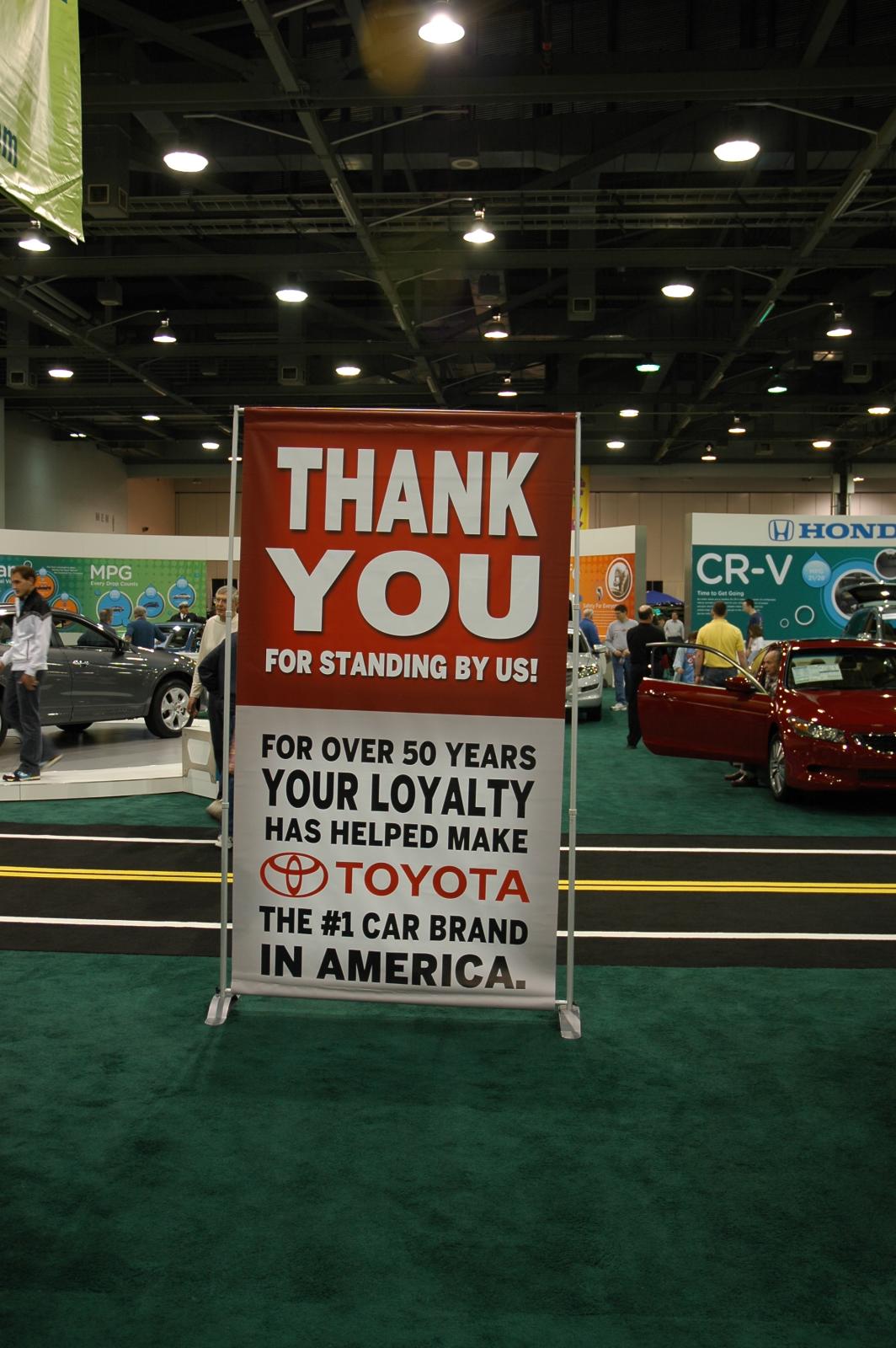This detailed image, taken at an indoor car show, captures the busy environment of an expo center with a black ceiling and factory lighting leading off into the distance. Green carpeting covers much of the area, segmented into two levels connected by three black steps marked with white and yellow lines. A prominent stand in the foreground features a red and white poster thanking loyal customers for making Toyota the number one car brand in America for over 50 years, emphasizing the words "thank you for standing by us."

Multiple cars are on display, including a teal Honda CR-V, identifiable by a large poster bearing the Honda logo situated behind it. Other vehicles include a red car on the right, a white car in the middle, and a gray car on the left, with various banners positioned behind them, one of which indicates "MPG." Some cars have open doors and window stickers, adding to the interactive appeal of the show. The image also captures several attendees either inspecting the cars closely or engaging with exhibitors, further highlighting the vibrant atmosphere of the event.